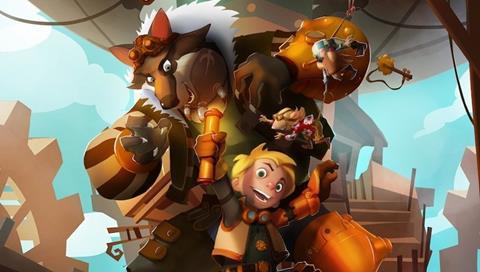The illustration is a vibrant, cartoony scene featuring a whimsical ensemble of steampunk characters in the center. Dominating the scene is a large steampunk wolf-like creature with blue eyes and cog-covered goggles, wearing a large furry coat and metal gauntlets. The creature appears to be trying to snatch a glowing, golden map from the hands of a small boy with wide eyes and a hysterical grin. The boy, dressed in a green shirt with cogwheel buttons, a vest, and goggles around his neck, holds the map aloft and looks directly at the viewer, seemingly unaware of the wolf's intention. Accompanying these characters are two mice – one hanging off the wolf’s arm and the other, wearing goggles and a red shirt, also reaching for the map. The backdrop features large, intricate gears and mechanical objects, as well as the bottom of a blimp, against a backdrop of blue sky and clouds, evoking a fantastical, steampunk atmosphere reminiscent of a children's movie or a mobile game advertisement.